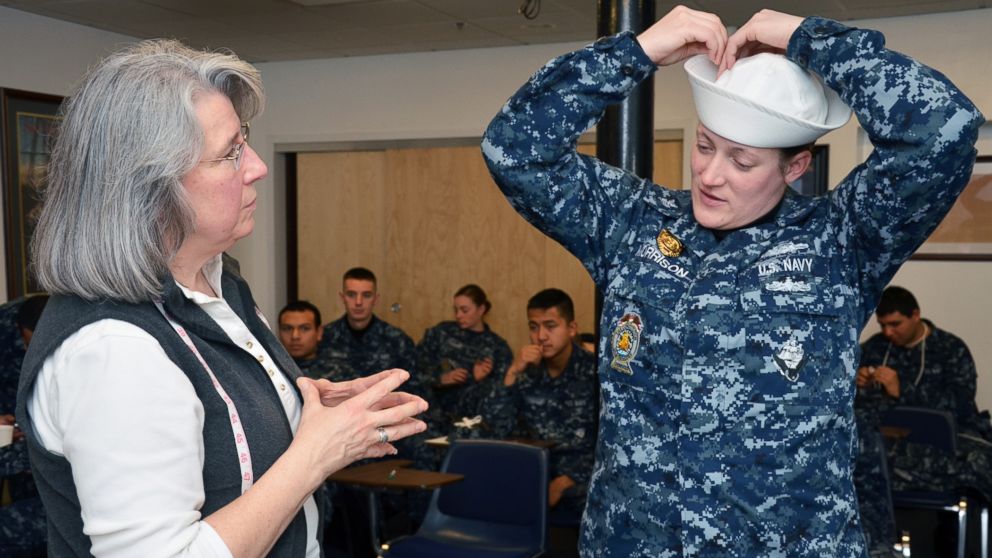In the image, a group of individuals is prominently featured in a military setting. In the background, at least five people are seated in rows, all dressed in black and gray camouflage uniforms. The group consists of four men, identifiable by their short hair, and one woman, with her hair neatly tied back. The scene is set against wooden doors and a white wall, with a desk featuring a brown tabletop and a blue chair adding to the composition.

In the foreground, the profile of a woman captures attention. She is dressed in a white shirt layered under a black vest, her shoulder-length gray hair framing her face. She wears glasses and has a ring on the third finger of her right hand. The woman is intently observing another individual, who is attired in a camouflage outfit bearing the label "U.S. Navy." The individual's name tag is partially obscured by the fabric, making it unreadable. They are also wearing a white sailor's hat, which both of their hands are gently holding. The detailed elements of their attire and surroundings hint at a formal military event or assembly.